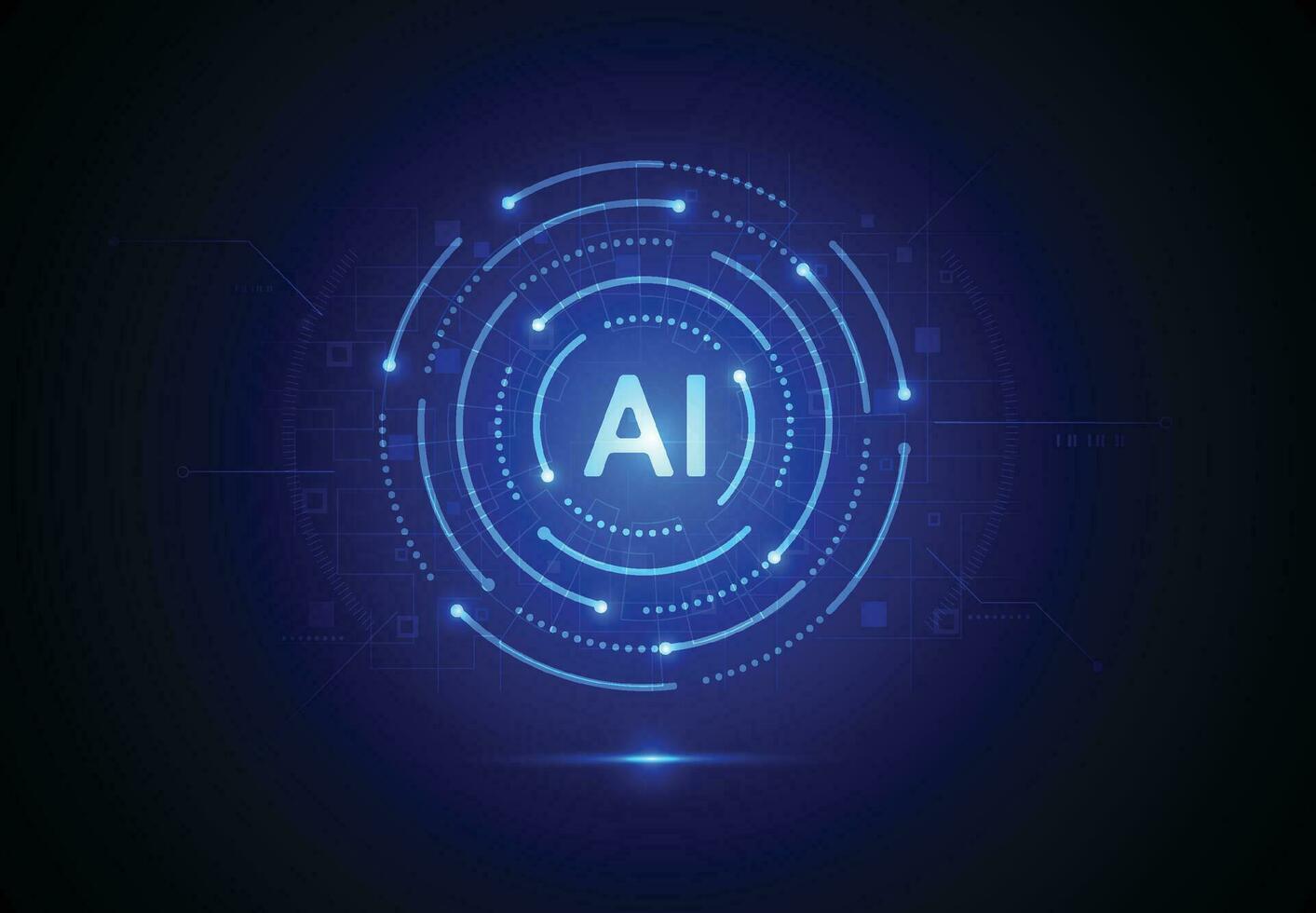The image depicts a visually striking, futuristic graphic reminiscent of radar or sonar displays, set against a completely black background. Radiating from the center, five circular layers composed of broken lines and bold white dots gradually fade from white to a deep navy blue as they extend outward, giving the circles an incomplete, segmented appearance. At the very center, the letters "AI" are prominently displayed, with a soft, white-to-light-blue gradient emanating from the core. These elements create the illusion of light emerging from the letters and the concentric circles, adding depth and a dynamic presence to the composition. The overall effect suggests a high-tech, data-driven visualization, potentially serving as a slide in a presentation about artificial intelligence.